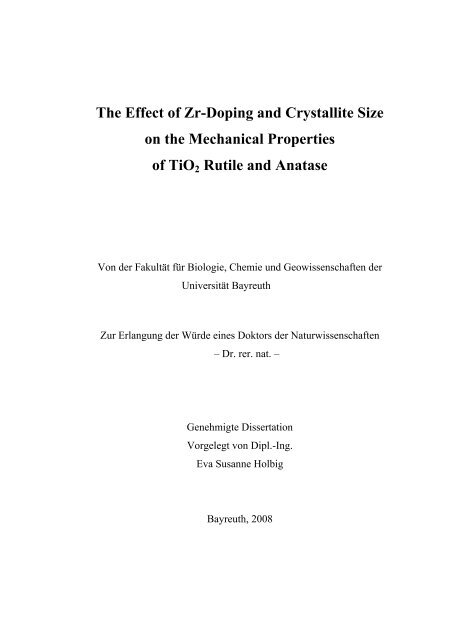The image is a page featuring black text on a white background. At the top, a bold black title reads, "The Effect of Zr-Doping and Crystallite Size on the Mechanical Properties of TiO2 Rutile and Anatase." Below this, there are two lines in German: "Naturwissenschaftliche Fakultät der Universität Bayreuth," and "Zur Erlangung der Würde eines Doktors der Naturwissenschaften vorgelegte Dissertation," followed by "Vorgelegt von Dipl.-Ing. Eva Susanne Holbig." The page concludes with "Bayreuth 2008" at the bottom.